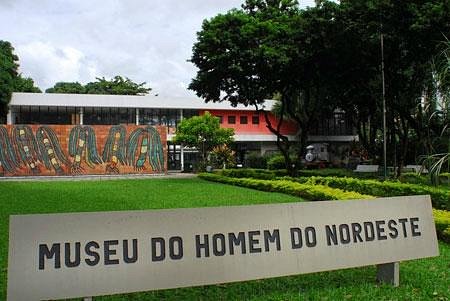The image is a color photograph taken outdoors during a cloudy day. It is in landscape orientation and captures a building set against a sky filled with light gray clouds. Dominating the bottom of the image is a low, rectangular gray plaque displaying the black text "Museu do Homem do Nordeste." 

In the background, the main subject is a large, salmon-colored building with a long white roof. This two-story structure features a blend of architectural materials, predominantly large windows interspersed with sections of brick, especially noticeable on the left and far-right sides. 

In front of the building, there is a painted brick wall adorned with an abstract mural depicting striped poles that resemble palm trunks with long, greenish-blue fronds or leaves descending from the top. 

To the right, several mature trees with dark green leaves stand alongside a hedgerow lining a path that extends from the bottom right corner towards the center of the image, threading through a healthy, vibrant green lawn. Behind the building, additional trees with small, dark green leaves are visible, adding more depth to the scene. The style of the photograph leans towards realistic representation, capturing the detailed elements of this outdoor setting.